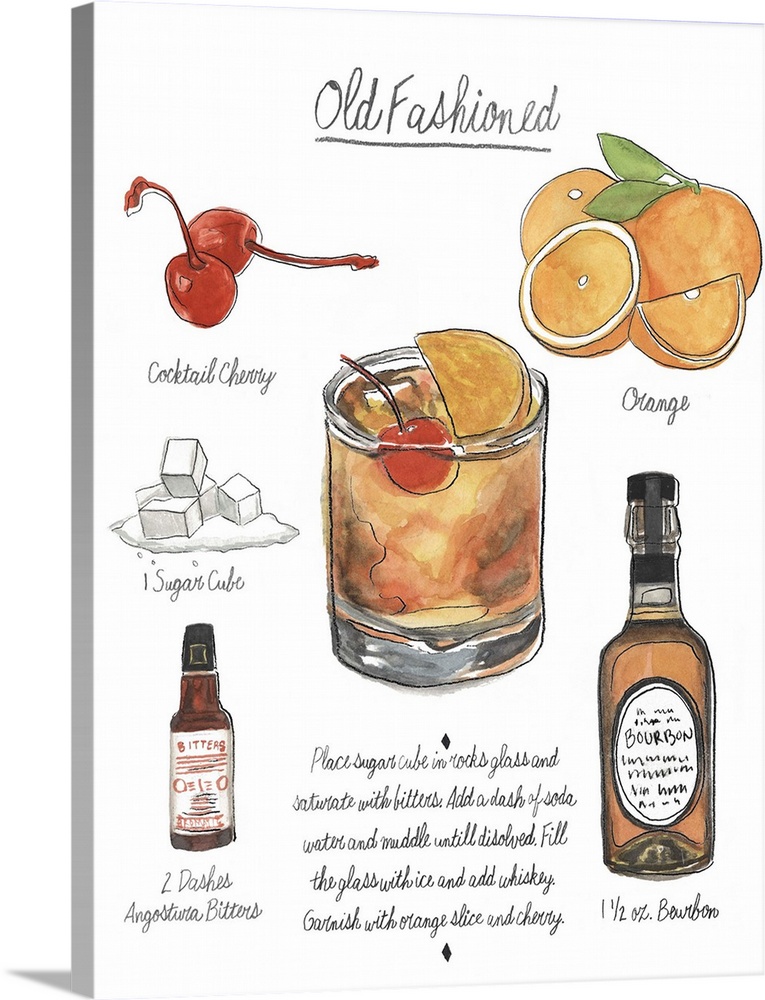This poster illustrates the recipe for making an old-fashioned cocktail in a detailed, hand-drawn style. At the top left, there's a sketch of two maraschino cherries labeled "cocktail cherry." On the top right, an illustration displays two whole oranges, a half orange, and a quarter orange with the label "orange." On the left side of the mid-section, four sugar cubes are stacked on a pile of granulated sugar, labeled "one sugar cube." Centrally placed is an image of the final old-fashioned cocktail in a clear glass, garnished with a cherry and a slice of orange. The top-right section features a group of oranges, labeled "orange." On the bottom right is a drawing of a bourbon bottle with the word "bourbon" prominently displayed on the label. Accompanying this image are the measurements "one and one-half ounce of bourbon." On the bottom left, there's a bottle labeled "Angostura bitters" with text below stating "dashes of Angostura bitters." Below this, the largest graphic on the poster provides the step-by-step instructions: "Place sugar cubes in rocks glass and saturate with bitters, add a dash of soda water, and muddle until dissolved. Fill the glass with ice and add whiskey. Garnish with an orange slice and a cherry."